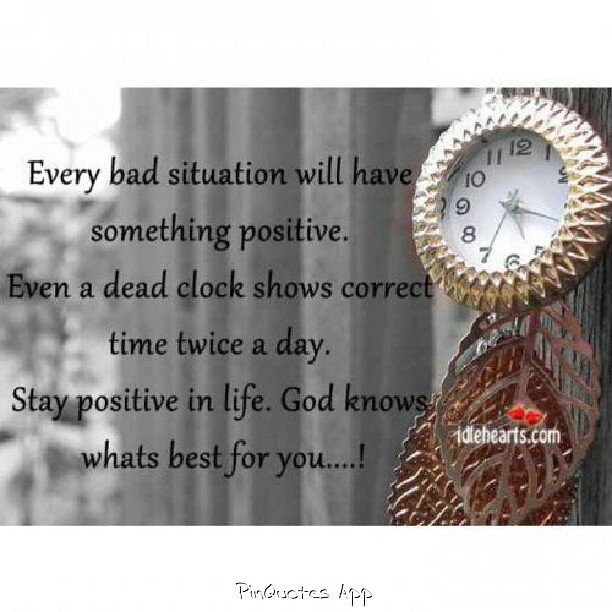The image is a digitally rendered, inspirational photo with a mixed black-and-white and colored scheme. On the right-hand side, there's a decorative clock adorned with a gold rim, a white face, and black numbers. Below the clock, there are intricately designed leaves that appear to be made of copper or metal, adding a touch of color to the otherwise monochromatic background. The main text, written in black and positioned on the left and center, reads: "Every bad situation will have something positive. Even a dead clock shows correct time twice a day. Stay positive in life. God knows what's best for you......!" Below this text, on one of the metallic leaves, the watermark 'idlehearts.com' is inscribed. Additionally, at the very bottom of the image, against a white background, the text 'Pin Quotes App' is visible.